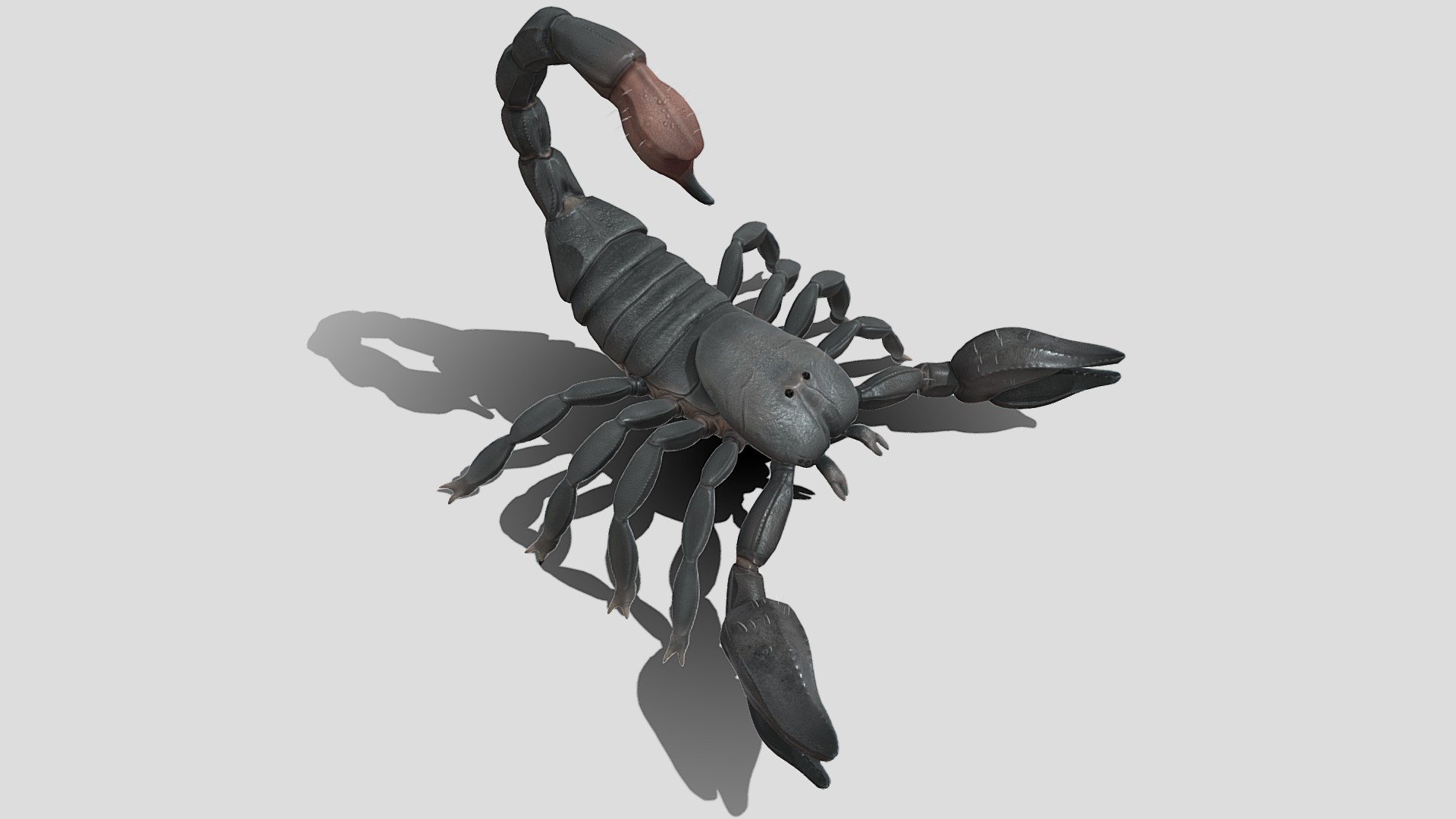The image features a detailed 3D-rendered model of a slightly cartoonish scorpion that resembles a sculpture or a piece of artwork. It appears to be made of a material that could be metal, plastic, or clay, characterized by a metallic or ribbed texture. The scorpion is predominantly light gray with some dark gray and brown accents, particularly on the stinger at the end of its curled tail. The body is segmented with ridges, and it has notable features including unusually shaped, rounded pinchers at the front, eight jointed legs that curl underneath, and two small black beady eyes atop its head. The model is situated on a flat, light gray background, and a strong light source from above casts a detailed shadow beneath it, adding depth to the overall presentation. The image is cropped horizontally, focusing closely on the scorpion facing the bottom right-hand corner, highlighting its intricate design and texture.